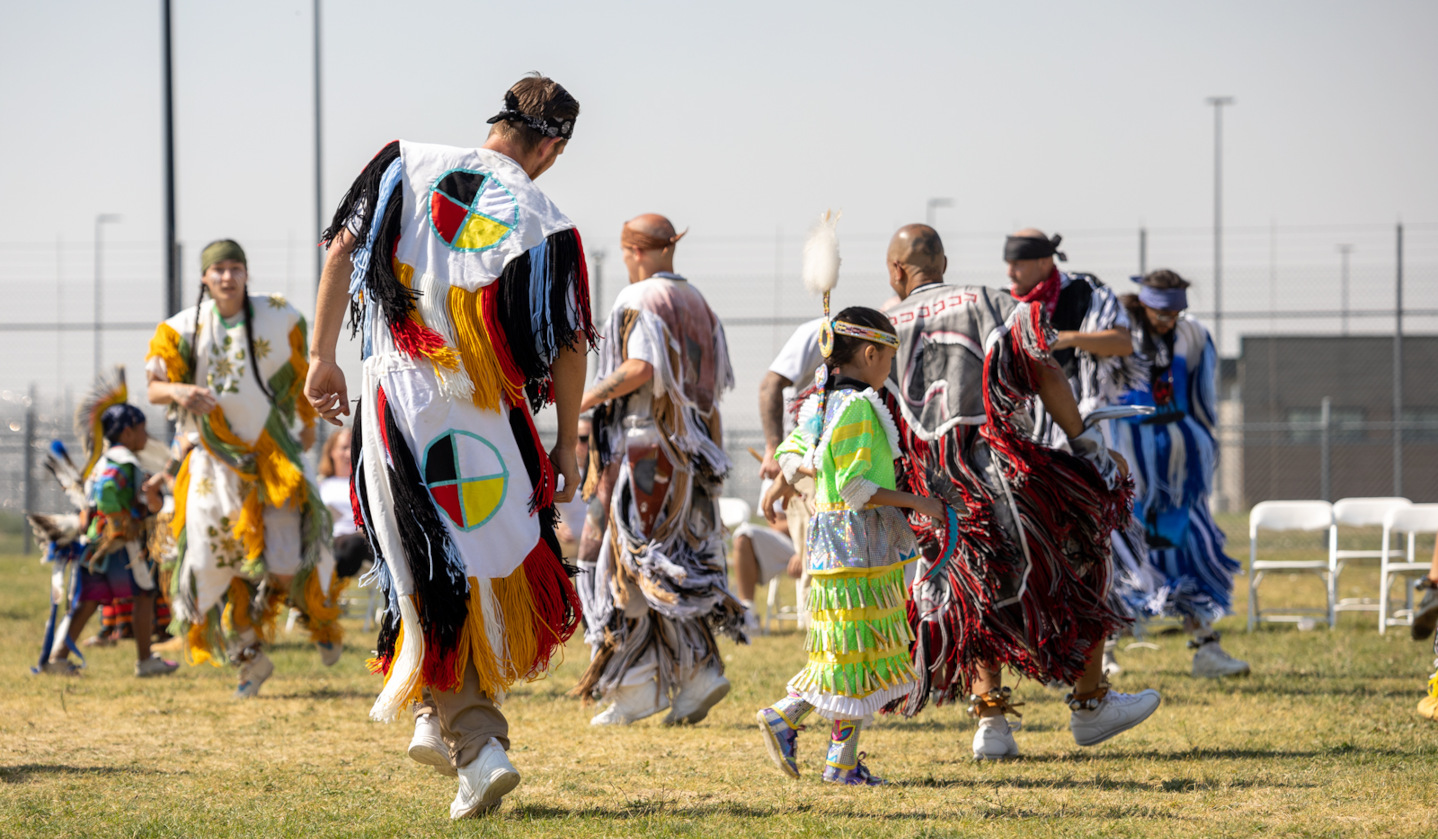The image captures a vibrant scene of a Native American festival on a bright sunny day, set in an open grassy field with most of the grass appearing brown. The group, consisting of about six to seven adults and a few children, are dressed in traditional, brightly colored attire adorned with various designs and fringes. The adults and children seem to be engaged in a traditional dance, their movements captured mid-action, giving the impression of a lively celebration. All participants wear headbands instead of headgear, with one adult distinguished by long braids and a robe decorated in yellow, green, and white. Another adult's robe features red, black, and gray patterns, while a young person is notably dressed in green and yellow with a silver midsection. The colorful garments include shades of blue, white, mustard yellow, olive green, red, and black, each embellished with unique fringe decorations. White folding chairs are visible to the side, and a metal fence along with poles, possibly for streetlights, are present in the background, suggesting this is a well-organized community event. The festive and communal atmosphere is palpable, with everyone immersed in the cultural dance.